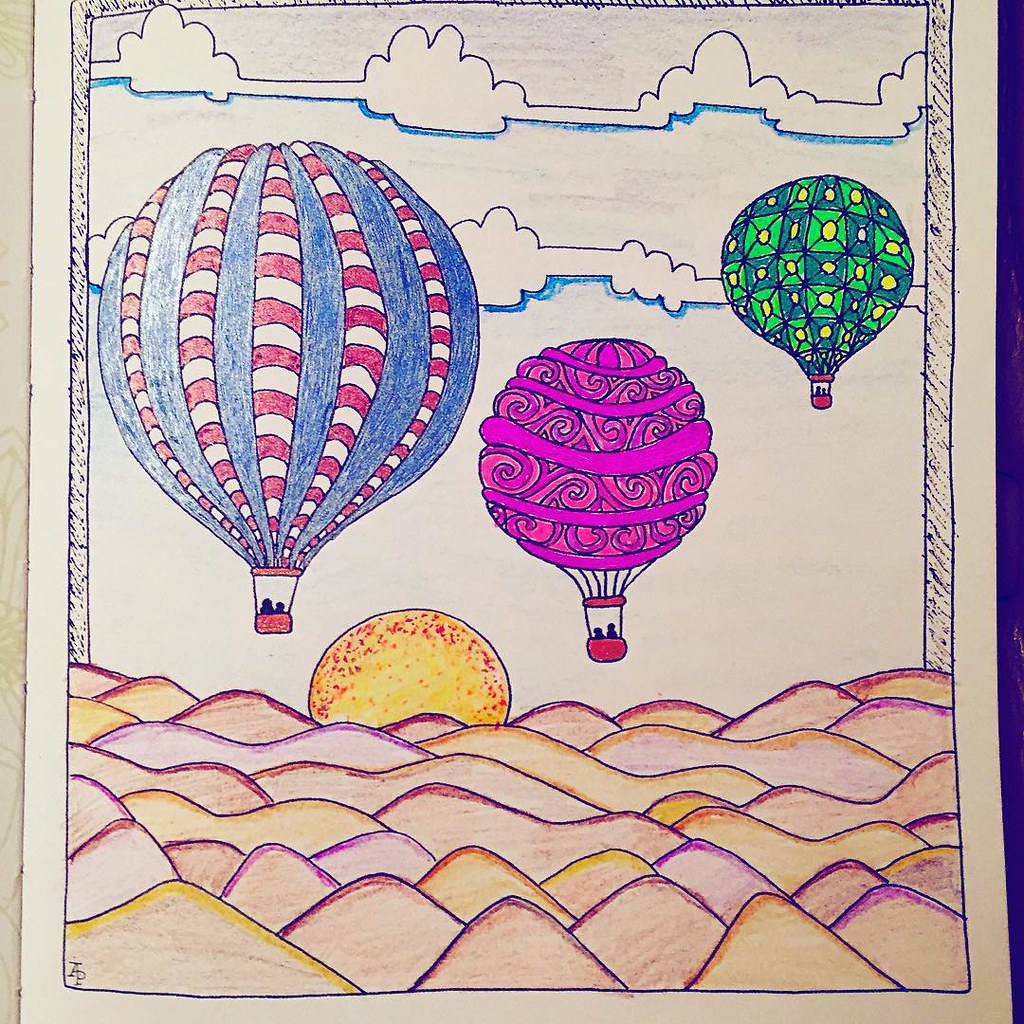This image depicts a vibrant scene of three hot air balloons, each distinctly colored and detailed, seemingly floating across a tranquil desert landscape during either sunrise or sunset. The balloons, hand-colored using crayons or colored pencils, vary in size and design. One balloon features blue with red and white stripes; another is adorned with purple swirly designs; and the third displays green squares with yellow circles. Each balloon has a red basket at its base, housing the silhouettes of two people. Below them, the rolling sandy hills display an array of purples, yellows, and oranges, while the sky above is a serene blue with scattered clouds. A radiant yellow sun with orange and red accents is positioned low on the horizon, casting a warm glow over the entire scene.